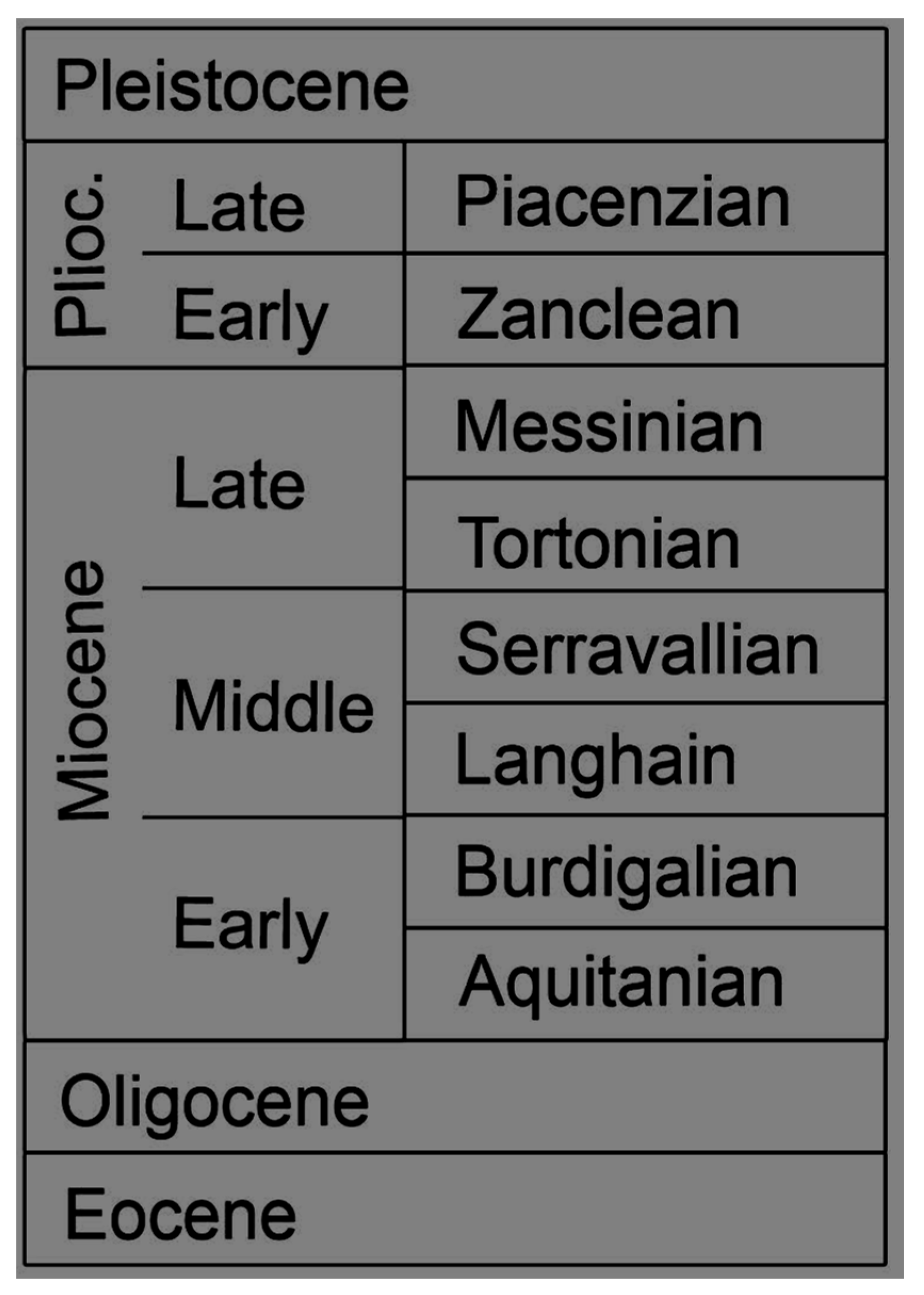The image displays a detailed black and white table, likely from a geology textbook, outlining different geological time periods and their subdivisions. The top of the table is headed by the word "Pleistocene." Below it, the table is divided into columns, with one column prominently featuring sideways-aligned text, possibly abbreviations. The first main section is labeled "Pliocene," abbreviated as "Plioc.," and is further divided into "Late Piacenzian" and "Early Zanclean." The next category is "Miocene," split into "Late Miocene" (Messinian and Tortonian), "Middle Miocene" (Serravallian and Langhian), and "Early Miocene" (Burdigalian and Aquitanian). Following these are rows for "Oligocene" and "Eocene." The table has a simple, close-up view with dark gray paper and black text.